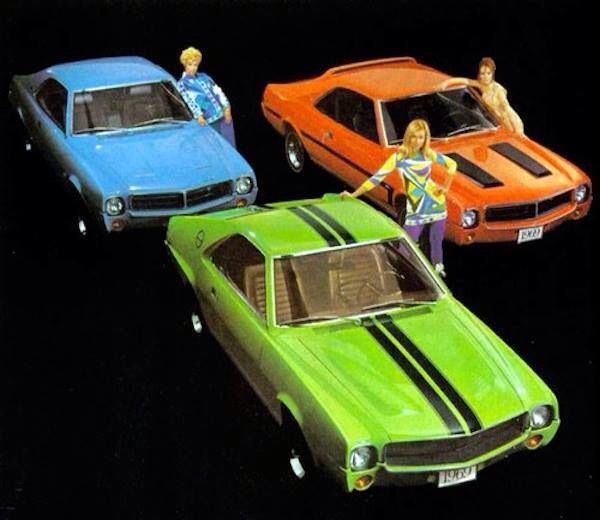This image showcases three vintage sports cars from the late 1960s or 1970s, set against a stark black background. Each car is paired with a woman dressed in colors that complement the vehicles. In the foreground center, there is a lime green car with two black stripes running over the hood, roof, and trunk. Its interior is tan, and standing next to it is a blonde woman dressed in purple leggings and a tunic adorned with a vibrant mosaic pattern in blue, purple, yellow, green, and black. To the right, partially behind the green car, is a striking orange sports car with black detailing. A red-haired woman, wearing a tan dress, leans gracefully over the roof of this car. To the back left of the image, we see a baby blue sports car. A blonde woman with short hair, dressed in blue pants and a blue and white patterned shirt, stands beside this vehicle. The overall composition and colors give the scene a nostalgic yet dynamic feel, emphasizing the style and elegance of the era.